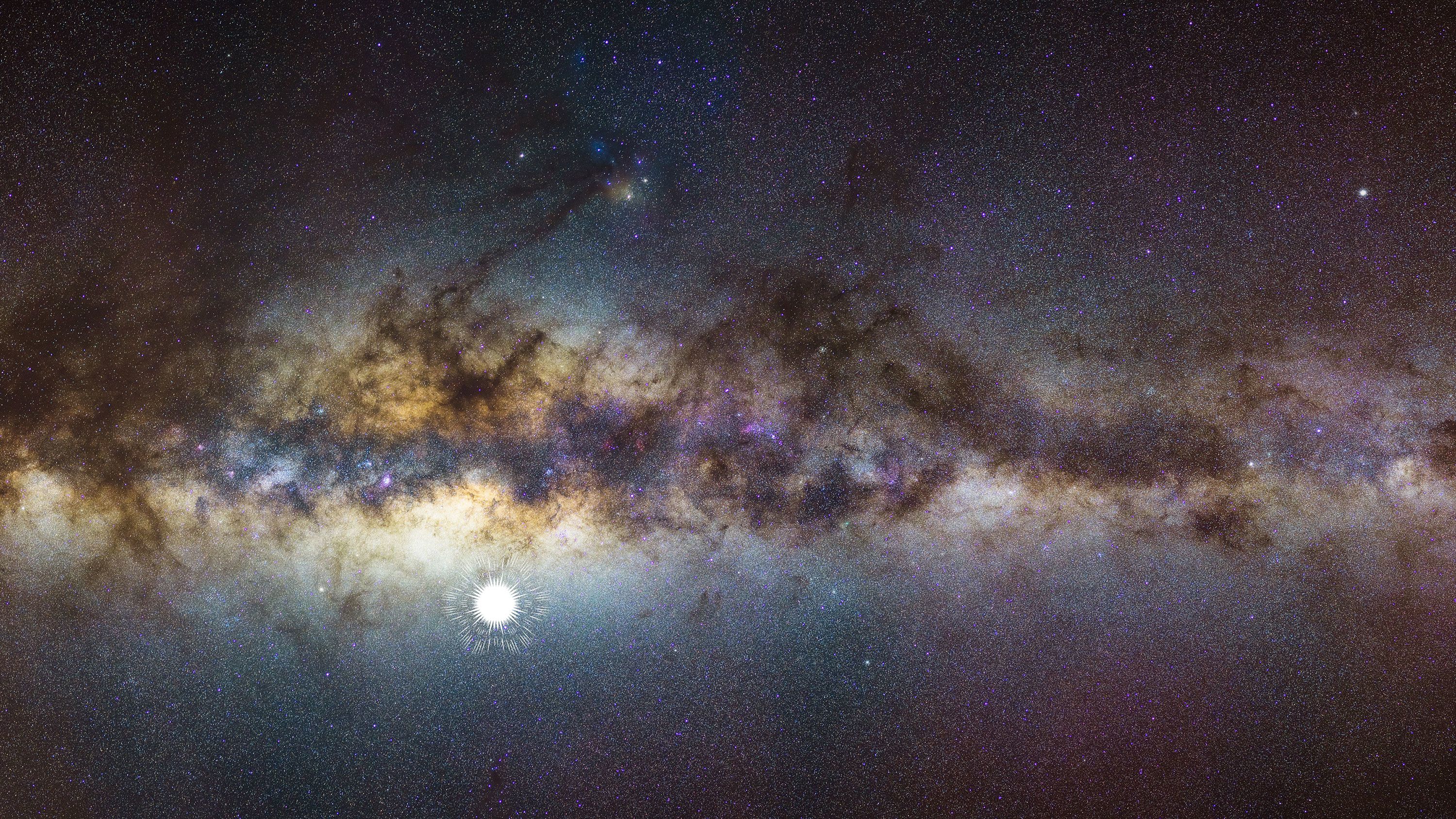This captivating image, likely captured by a deep space telescope, showcases the awe-inspiring vastness and beauty of a faraway galaxy. Dominating the center of the photograph is a luminous band resembling the Milky Way, adorned with a myriad of celestial colors including white, yellow, purple, dark brown, light purple, and light blue. A striking, bright white star with small protruding rays can be seen near the bottom left, standing out against the darker background. The corners of the image transition from deep black to dark blue, further enhancing the depth and mystery of space. As your gaze moves upward, the galaxy's intricate patterns gradually fade into a deep, space-black backdrop. Millions of tiny stars dot the top portion of the photograph, creating a stunning contrast against the dark expanse, and conveying the immensity of the cosmos.